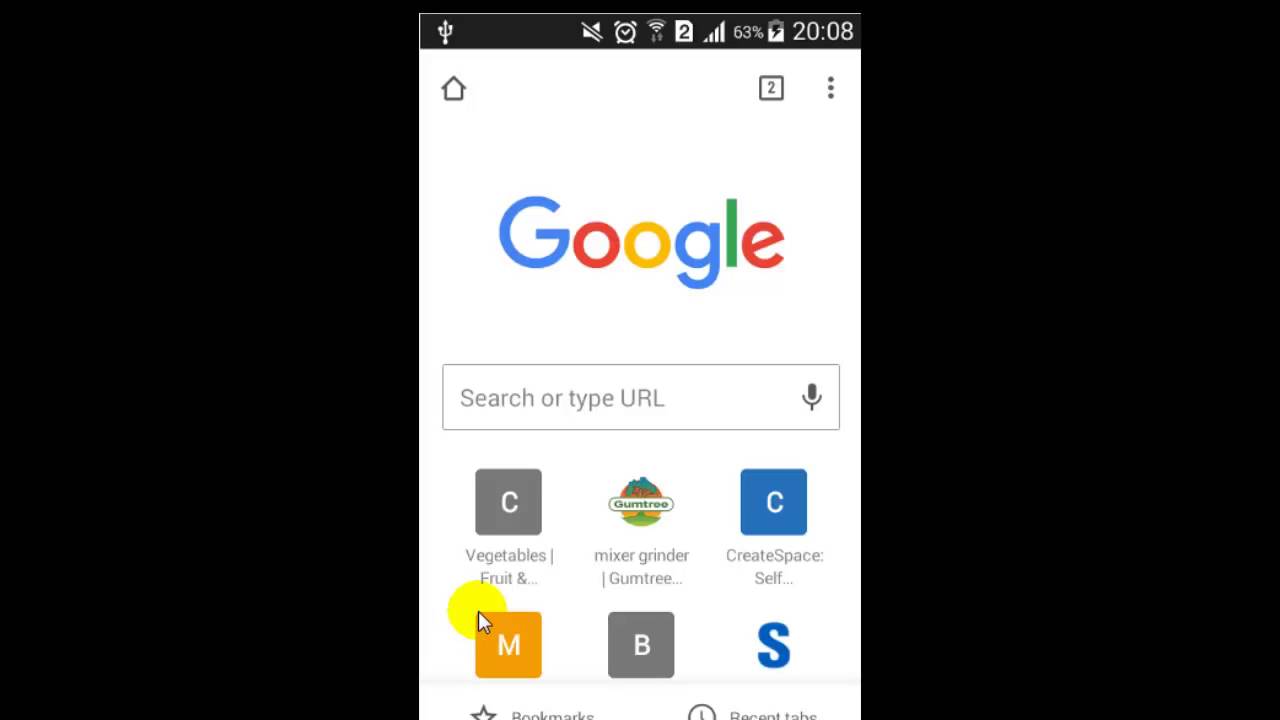The image showcases the interface of a digital device, likely a smartphone, featuring the Google homepage. At the very top right corner, the time is displayed in white using a 24-hour (military) format, indicating "20:08." To the left of the time, the battery percentage is shown at 63%, accompanied by the battery icon. Further to the left, signal bars indicate the phone's network connectivity, followed by four additional icons: a number "2," a Wi-Fi symbol, a clock symbol, and a mute symbol (a speaker with a slash through it).

The top section, containing these icons, is set against a black background, contrasting with the rest of the image which has a white background typical of the Google homepage. Centrally located, the colorful Google logo is displayed, with the letters in blue, red, yellow, and green. Above the logo, on either side, are the home icon on the left and a box with the number "2" followed by three dots on the right.

Below the Google logo is a search bar labeled "Search or type URL," featuring a speaker icon for voice input. Further down, there are six distinct boxes, suggesting quick-access functions or bookmarks.